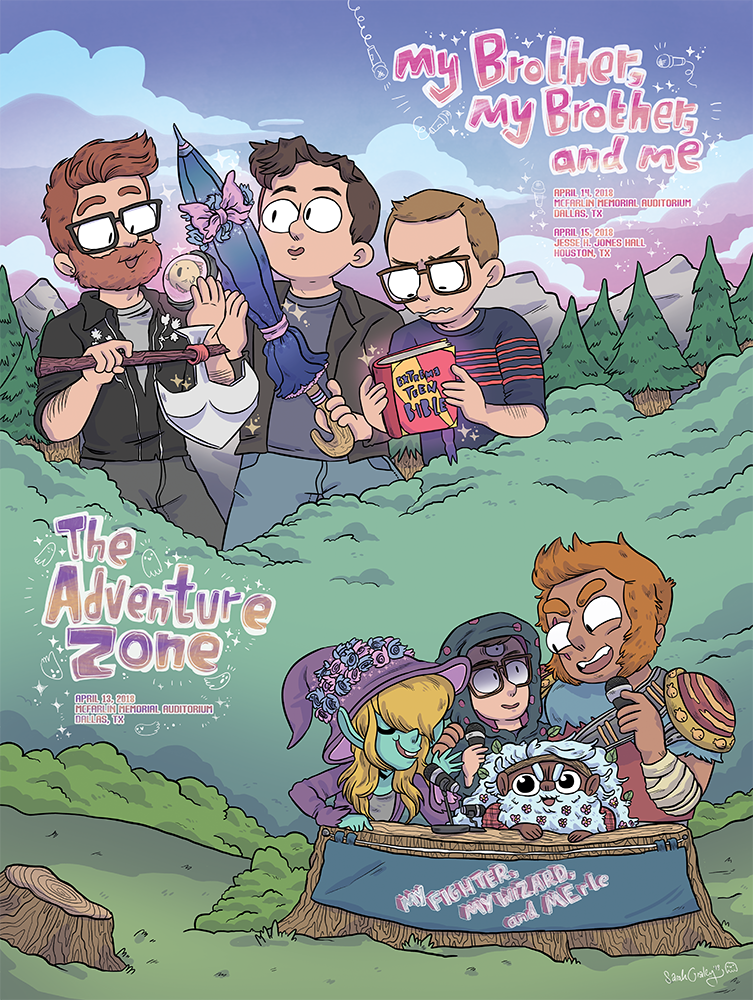The image appears to be a highly detailed, possibly computer-generated or hand-drawn poster promoting two events. The top section of the poster, adorned with a pink ombre background, features the title "My Brother, My Brother and Me" alongside event dates: April 14, 2018, at McFarland Memorial Auditorium in Dallas, Texas, and April 15, 2018, at Jesse H. Jones Hall in Houston, Texas.

Dominating the upper left area of the poster are three men, stylized in a cartoonish, Dungeons and Dragons-inspired art style. One man with a beard and brownish-red hair, wearing glasses, a black sweatshirt, dark gray jeans, and a gray t-shirt, is holding an axe. To his right, a brown-haired man sports a gray t-shirt, blue jeans, a brown jacket, and holds a purple umbrella with a pink bow. The third figure, a blonde man with glasses, wearing a black t-shirt with red stripes, holds a book titled "Extreme Teen Bible."

In the center, in a fun, colorful font of blue, purple, and orange, the words "The Adventure Zone" stand out, hinting at an adventurous, possibly fantasy-related event.

The bottom right corner introduces a secondary group of fantastical characters labeled "My Fighter, My Wizard, and Merle." This trio includes a green-skinned woman with blonde hair in a purple dress and wizard’s hat adorned with roses, a three-eyed man dressed in a black coat with red dots, and a small bearded man with white hair wearing a red plaid shirt with flowers in his beard. They stand behind a tree trunk, sharing the scene with a tiny troll-like creature and a fairy.

The background integrates a rich, natural landscape of mountains, trees, and a pink and purple sky, enriching the fantastical and captivating atmosphere of the poster, suggesting a promotional piece for a live show or podcast event celebrating fantasy themes and adventure.